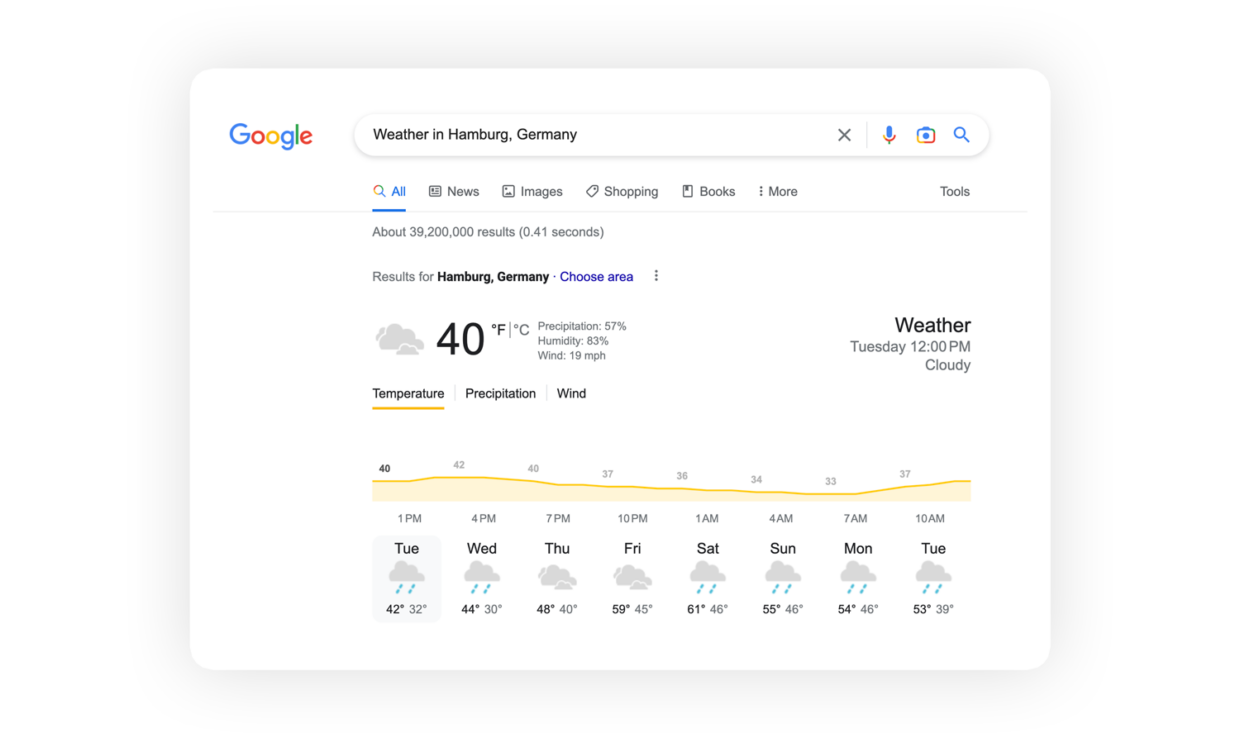A detailed Google search results page for the query "weather in Hamburg, Germany" is displayed. At the top, the search box contains the text "weather in Hamburg, Germany" alongside an 'X' symbol for clearing the search, a microphone icon for voice input, an image icon, and a magnifying glass icon for initiating the search. Beneath the search bar, a variety of tab options are available, including "All," "News," "Images," "Shopping," "Books," "More," and "Tools." The page indicates about 39,200,000 search results were found in approximately 0.41 seconds.

Directly under this information, a weather summary is presented. A blue hyperlink reading "Choose Area" appears, followed by current weather conditions in Hamburg. The sky is depicted as cloudy, with a temperature of 40°F, precipitation at 57%, humidity at 82%, and wind speed at 19 mph. The detailed weather forecast begins at Tuesday 12 PM, showing cloudy conditions continuing through the day. Further detailed breakdown for the week includes:

- **Tuesday:** High of 42°F, Low of 32°F.
- **Wednesday:** High of 44°F, Low of 30°F.
- **Thursday:** High of 48°F, Low of 40°F.
- **Friday:** High of 59°F, Low of 45°F.
- **Saturday:** High of 61°F, Low of 46°F.
- **Sunday:** High of 55°F, Low of 46°F.